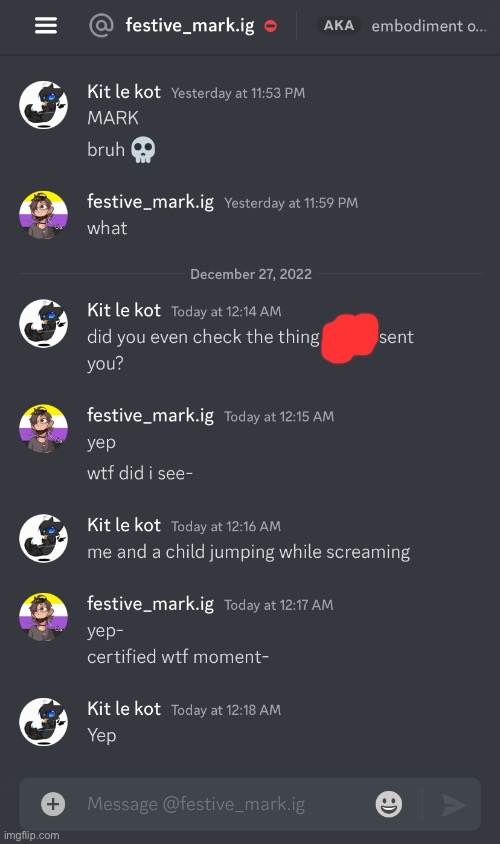Screenshot of an Instagram thread from user @festive_mark.ig, identified by a profile logo resembling a red stop sign with the username "aka embodiment." The thread captures a conversation between two users: Kit Lee Cat, whose avatar features a white logo with a black figure, and Festive Mark, whose avatar displays a cartoon person with a background of yellow, white, and purple stripes. 

In a chronological exchange:

- Kit Lee Cat initiates the conversation at 11:53 p.m. with "bra" and a skeleton emoji.
- Festive Mark responds at 11:59 p.m. with "what December 27th 2022."
- Kit Lee Cat follows up at 12:14 a.m., asking, "Did you even check the [blank]," where "blank" is censored with red paint.
- One minute later, Festive Mark replies, "yep WTF did I see."
- Kit Lee Cat answers at 12:16 a.m., describing a scene of "me and a child jumping while screaming."
- At 12:17 a.m., Festive Mark confirms with "yep certified WTF moment."
- The conversation concludes with Kit Lee Cat affirming with "yep" at 12:18 a.m.

Below the thread, the standard Instagram interaction features are visible: a text box for comments, an emoji menu, and a send button.